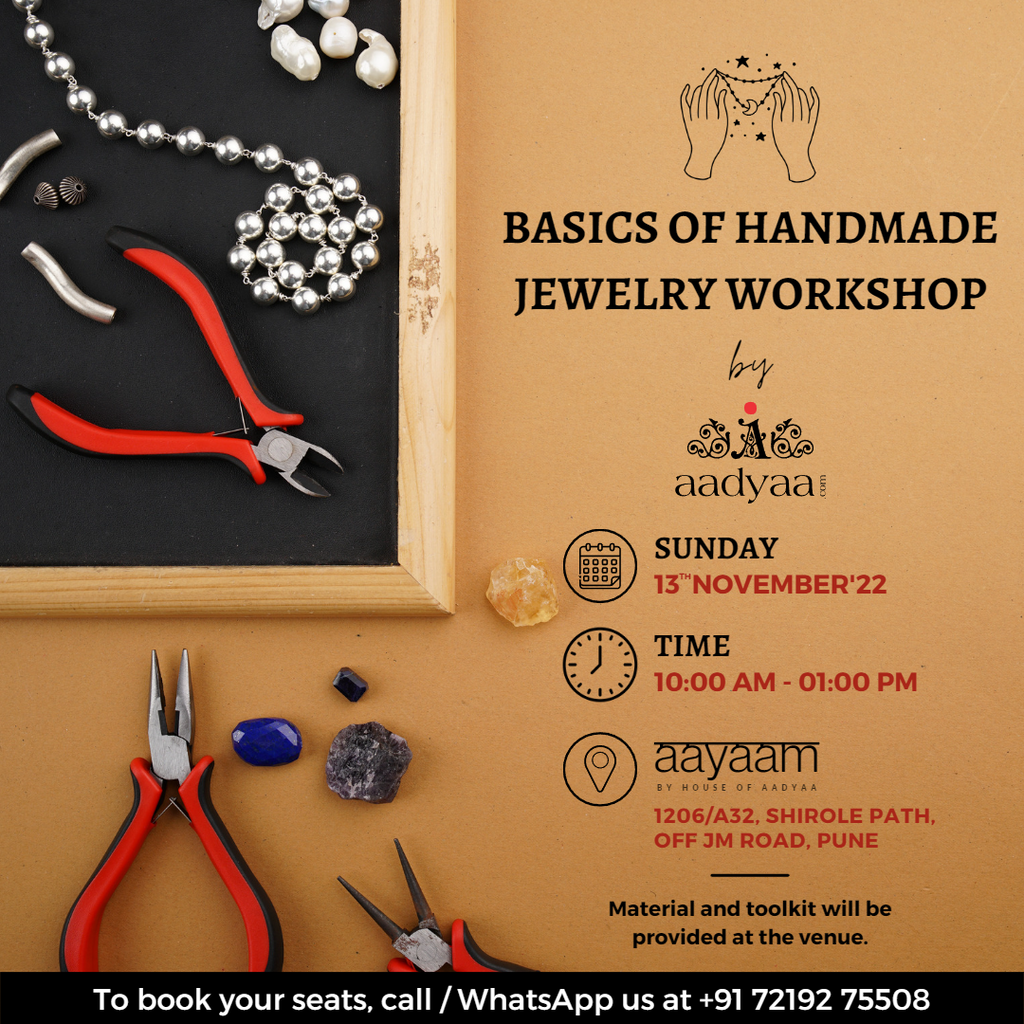The advertisement is set against a tan, yellowish-tan background. On the right side, there is a prominent image of hands holding a piece of jewelry adorned with a crescent moon and stars in black. Below this, "Basics of Handmade Jewelry Workshop" is printed in black font. Accompanying this text is a script logo featuring small leaves and an 'A' with an orange dot, followed by "A-A-D-Y-A-A" in lowercase letters. 

To the left, there is a framed board, possibly made of black felt bordered by light wood, displaying various jewelry-making tools and materials. These include a pair of red-handled pliers, a chain with silver balls, white shells in the top right corner, and metal pieces to the left.

To the right of the logo, details of the workshop are provided, reading: "Sunday, 13th November 2022" in red, with a calendar graphic and a clock face indicating the time "10 a.m. to 1 p.m." Below, in a black border, it states, "To book your seats, call or WhatsApp" followed by a phone number in white.

The event will be held at AAYAAM by House of Aadyaa, located at 1206 832 Sheroll Path, off JM Road, Pune. The workshop promises to provide materials and toolkits at the venue for participants.